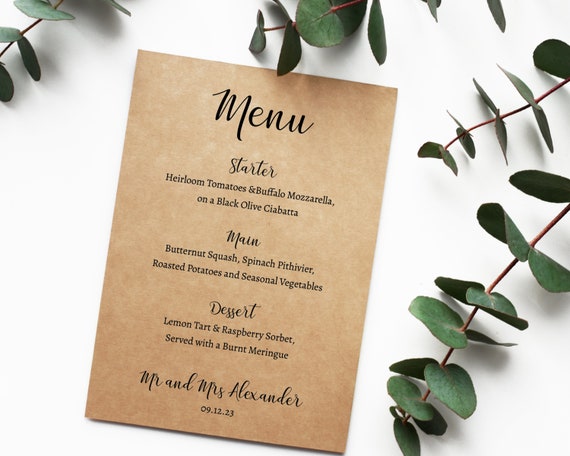The image captures a detailed photograph of a wedding menu centered on a white background, possibly a counter or table. The menu is a brown, cardboard-like card positioned at a slight angle. At the top, bold black letters spell out "Menu." Below this, the categories "Starter," "Main," and "Dessert" are listed sequentially, each followed by a specific dish: starter - heirloom tomatoes and buffalo mozzarella on a black olive ciabatta; main - butternut squash, spinach, pitchfewer, roasted potatoes, and seasonal vegetables; dessert - lemon tart and raspberry sorbet served with burnt meringue. The menu concludes with a personalized note, "Mr. and Mrs. Alexander 09-12-23." The setup is adorned with green leaves on brown stems surrounding the menu from the top and on the upper and lower right sides, adding an elegant touch to the white backdrop.